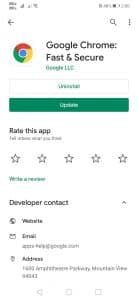Screen capture of a mobile app listing for Google Chrome on a smartphone, likely a Google Pixel. The app is described in the listing as "Google Chrome: Fast & Secure," with the iconic Google logo displayed beside it. The developer is noted as Google LLC. Below the app title, there are two prominent buttons: a white one labeled "Download" and a green one labeled "Update." The section below these buttons invites users to rate the app with a 5-star rating system and includes an option to write a review.

Further down the screen, in bold black text, is the option to contact the developer, offering links for the website, email, and a physical address. The image quality is notably poor and pixelated, making fine details difficult to discern. Despite this, the main function of the app, which is to browse the internet, is clear. The layout and design hint that the screenshot was likely taken from a Google Pixel device.